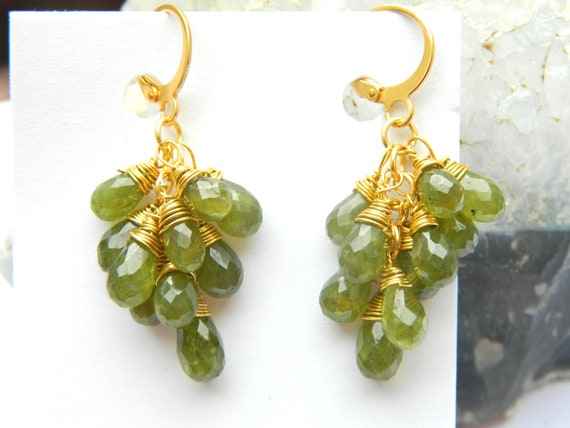In the image, a pair of dangling earrings is prominently featured, each meticulously attached to a white plastic or card-like holder, similar to the ones commonly found in stores. The earrings themselves are composed of gold-finished posts and chains that elegantly suspend an array of green, faceted gemstones. These gemstones, translucent and shiny, collectively form a cluster that closely resembles a bunch of green grapes. Each earring displays approximately eight of these grape-like formations, all connected to a central gold loop, creating a symmetrical and cohesive design. The background adds a contrasting element with a marbled appearance, transitioning from a white upper right corner to a predominantly black lower area with a small white section. This setting enhances the visual appeal of the earrings, making them stand out as both stylish and eye-catching.